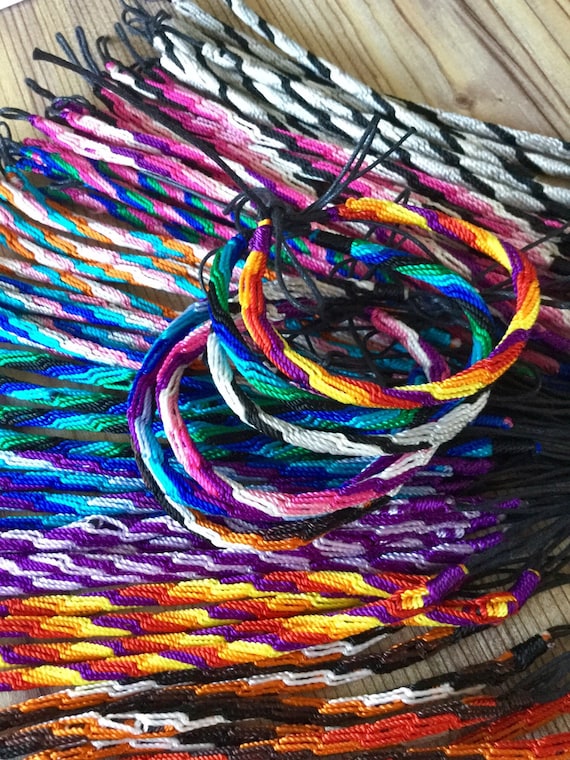The image shows an assortment of friendship bracelets arranged neatly on a wooden surface. The bracelets, crafted from woven thread, display a vibrant array of colors and patterns including black and white stripes, pink-white, purple and black stripes, pink-blue, green and purple stripes, white-orange, turquoise and white stripes, blue-green, blue-purple, purple-orange, red and yellow stripes, and brown, white and black stripes. Most of the bracelets are laid out flat, showcasing their colorful designs, while a few are already formed into bracelets, revealing how they look when worn. The wooden background contrasts with the bright hues of the bracelets, which are tightly clustered together, with some of their tying cords visible. The image composition highlights both the detailed patterns of each bracelet and the overall aesthetic of the collection.